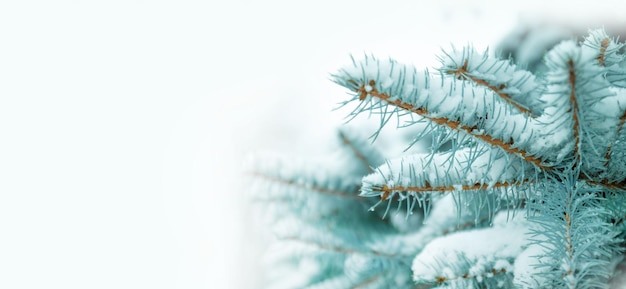This image captures the serene beauty of a snow-covered evergreen tree standing outdoors against a stark white background. The rectangular photograph, almost twice as long as it is tall, prominently features a cluster of branches from a Christmas tree-like evergreen, positioned mostly on the left side of the frame. The branches, heavily laden with snow, exhibit a unique bluish-green hue that contrasts strikingly with the pristine white snow, giving the snow a subtle tint. Clearly evident are the brown stems of the branches, with each needle encrusted in a layer of snow, some branches coated even more densely than others. Although a piece of the pale blue sky peeks out from the top, the main focus remains on the detailed, snow-laden branches that stretch out distinctly. The background appears intentionally blurred, emphasizing the intricate and frosty beauty of the evergreen, making the scene both tranquil and visually compelling.